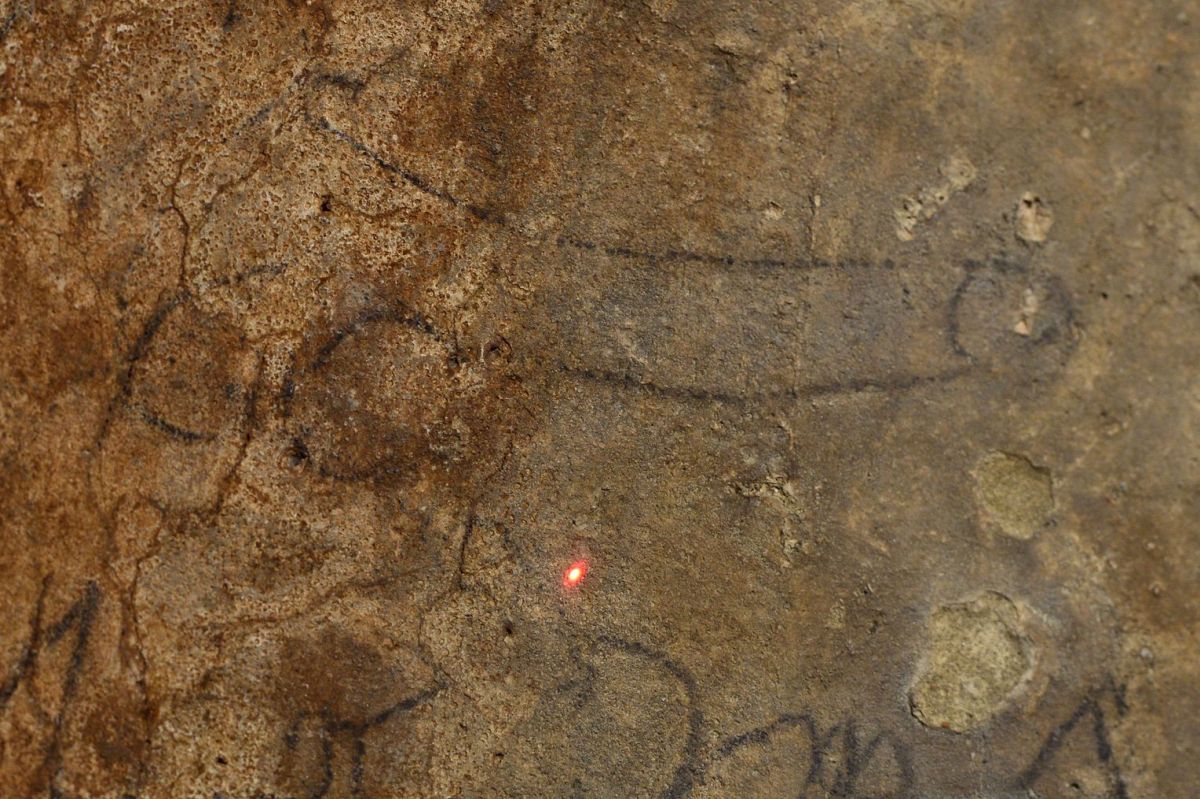This photograph captures a cave wall adorned with various shades of earthen colors—ranging from orange-brown to gray-brown—and appears weathered and worn, indicative of its ancient nature. In the bottom middle section of the wall, a red laser is seen shining on the surface, illuminating the crude graffiti. Predominantly drawn in black marker or charcoal, and appearing phallus-shaped with distinct wheels and resembling the Oscar Mayer Wienermobile, the prominent drawing seems created by a child or an inexperienced hand. Besides, there are abstract shapes, including two circle-like forms that might represent eyes, and other ambiguous shapes such as humps and a triangle, suggesting a mix of primitive art forms and childlike graffiti.